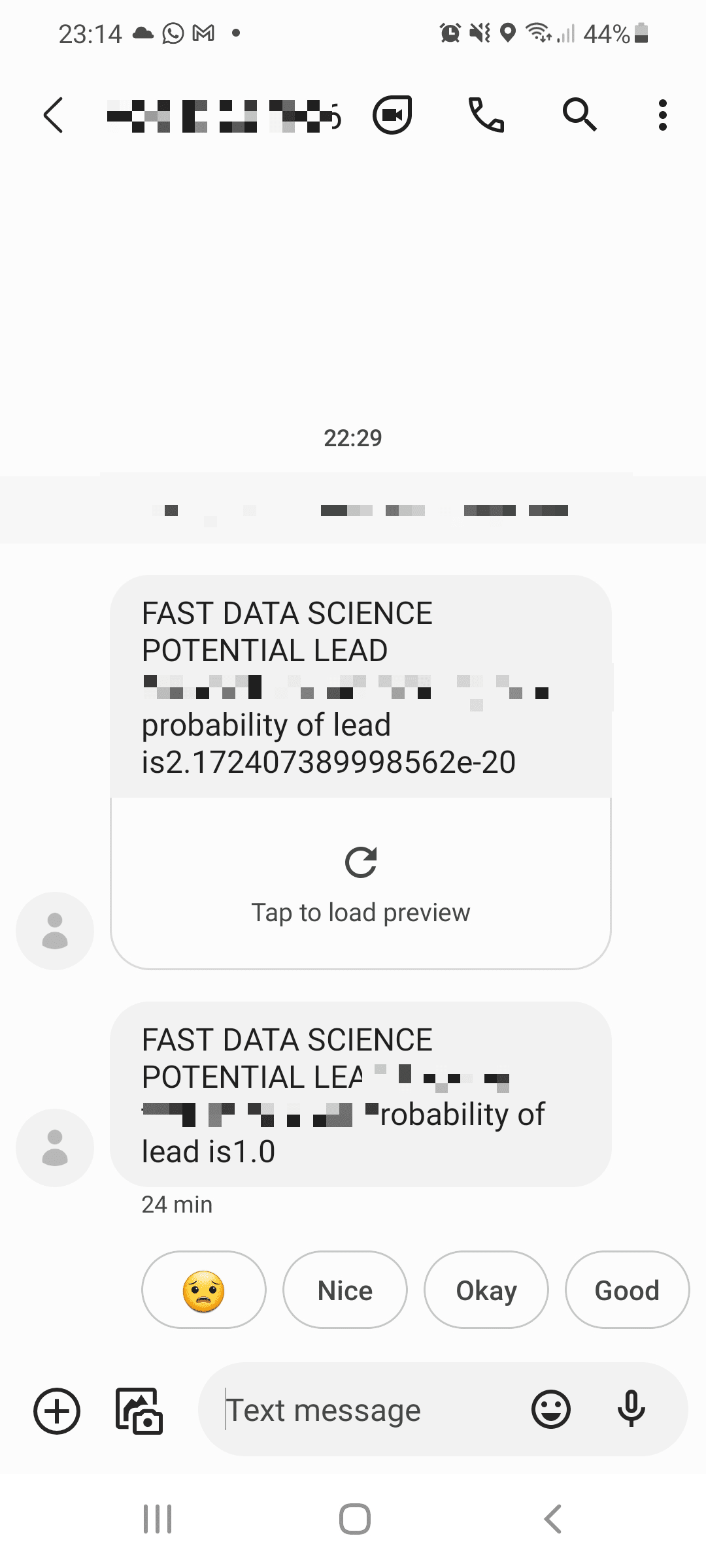The image displays a mobile phone screen with a website open, showcasing familiar icons and navigation elements. There is notable distortion across parts of the screen, characterized by black and white boxes, likely obscuring sensitive information. At the top of the screen, there is a search bar and a set of three dots representing a menu. Another element includes a black box with a circle around it. The time displayed is inconsistent, with one part showing 22:29 and another showing 23:14.

The primary content of the screen pertains to "Fast Data Science," indicating a "potential lead" with the probability of the lead obscured by the distortion. A lengthy number follows, accompanied by an option to "tap to load the preview." Repeat elements reappear mentioning "Fast Data Science" and "potential LEA," likely referring again to a lead, with a probability of 1.0 noted, though the 'P' in "probability" is somehow blacked out. The timestamp indicates this information was updated 24 minutes ago.

Below this information, there is an icon of a neutral-toned face, with descriptive words such as "nice," "okay," and "good." Further options on the screen include sending a text message, an emoji, or using a microphone feature to record a voice message.